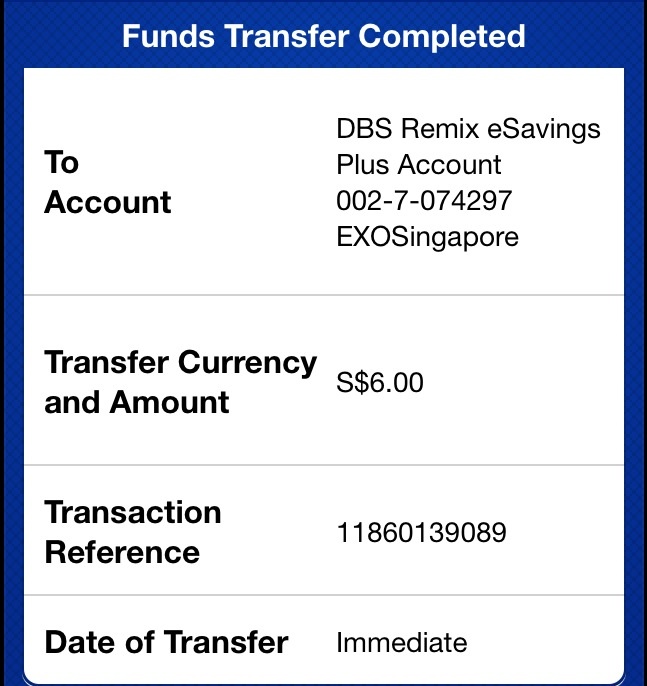The image depicts a digital receipt or screenshot from a financial app displaying a recently completed funds transfer. The screen features a blue background with a large white text box covering most of the area. At the top, in white text set against the blue background, it states "Funds Transfer Completed." Below this, within the white text box, there's detailed information structured in black text with light gray lines separating each section.

The receipt indicates the transfer is to a "DBS Remix eSavings Plus Account" with the account number "002-7074-297-EXO Singapore." It mentions the transfer currency and amount as "S$6.00" (Singapore dollars). A transaction reference number is provided: "11860139089." Lastly, it specifies that the date of the transfer is "Immediate." The left-aligned text is bolded, while the corresponding details on the right are not bolded.